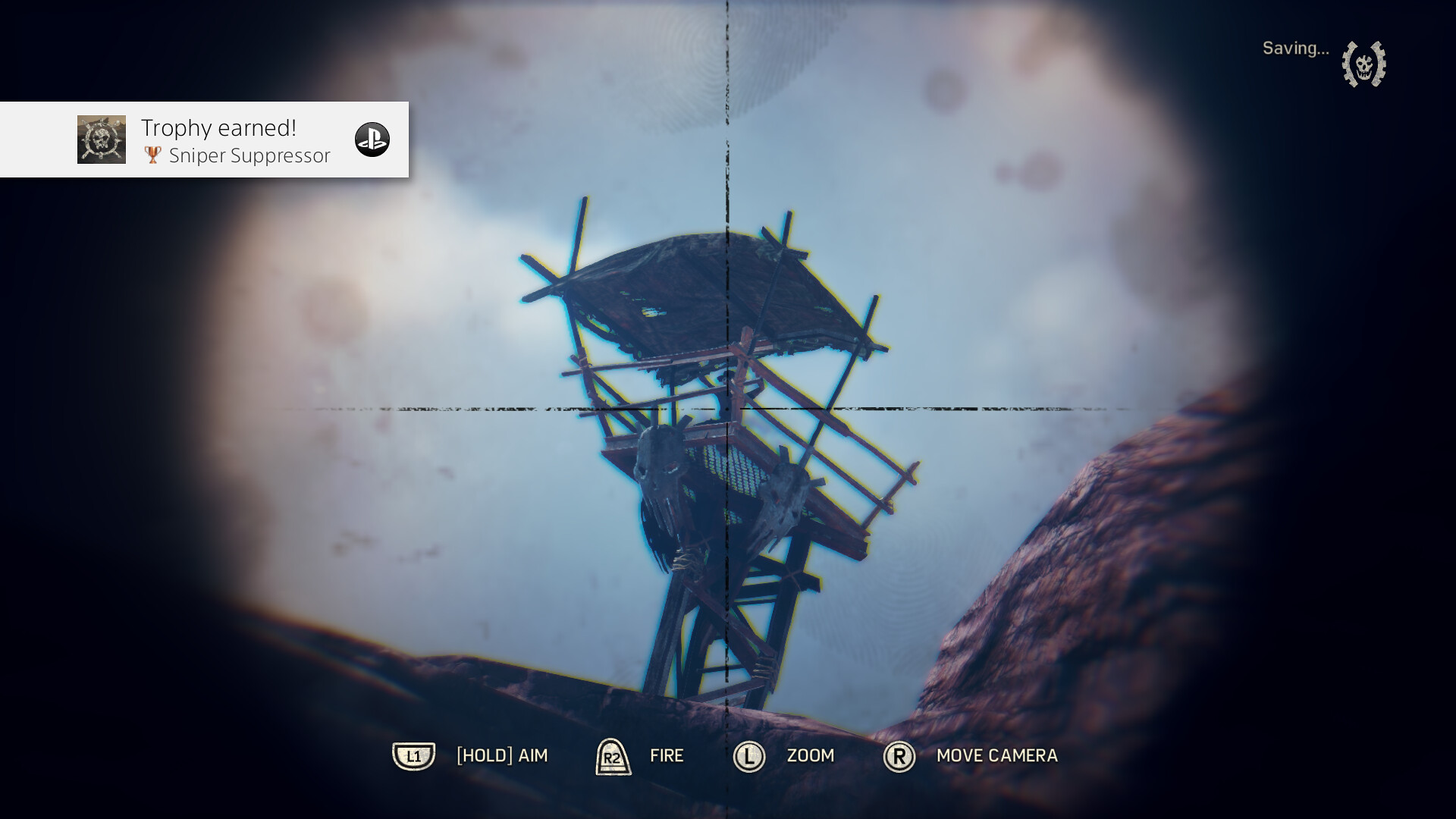This image is a detailed screenshot from a video game, captured through the perspective of a sniper scope. The corners of the image are blackened, simulating the view through a periscope. At the top left corner, there’s a white banner with light gray text that reads "Trophy Earned: Sniper Suppressor," accompanied by the PlayStation logo in red and a black circle with white lettering. Adjacent to the banner is an emblem featuring a skull in a circle. On the top right, the word "Saving" is displayed, with a badge of leaves curving around it. The central focus of the image is the sniper scope, with its crosshairs trained on a target located in a makeshift wooden sniper tower situated among red rocks under a blue sky. Cloud patterns can be seen in the background. Text overlays at the bottom of the image display game controls: "Hold", "Aim", "Fire", "Zoom", and "Move Camera," with L1, R2, the left stick, and the right stick respectively assigned to these actions. The backdrop shows part of a landscape that includes mountains.